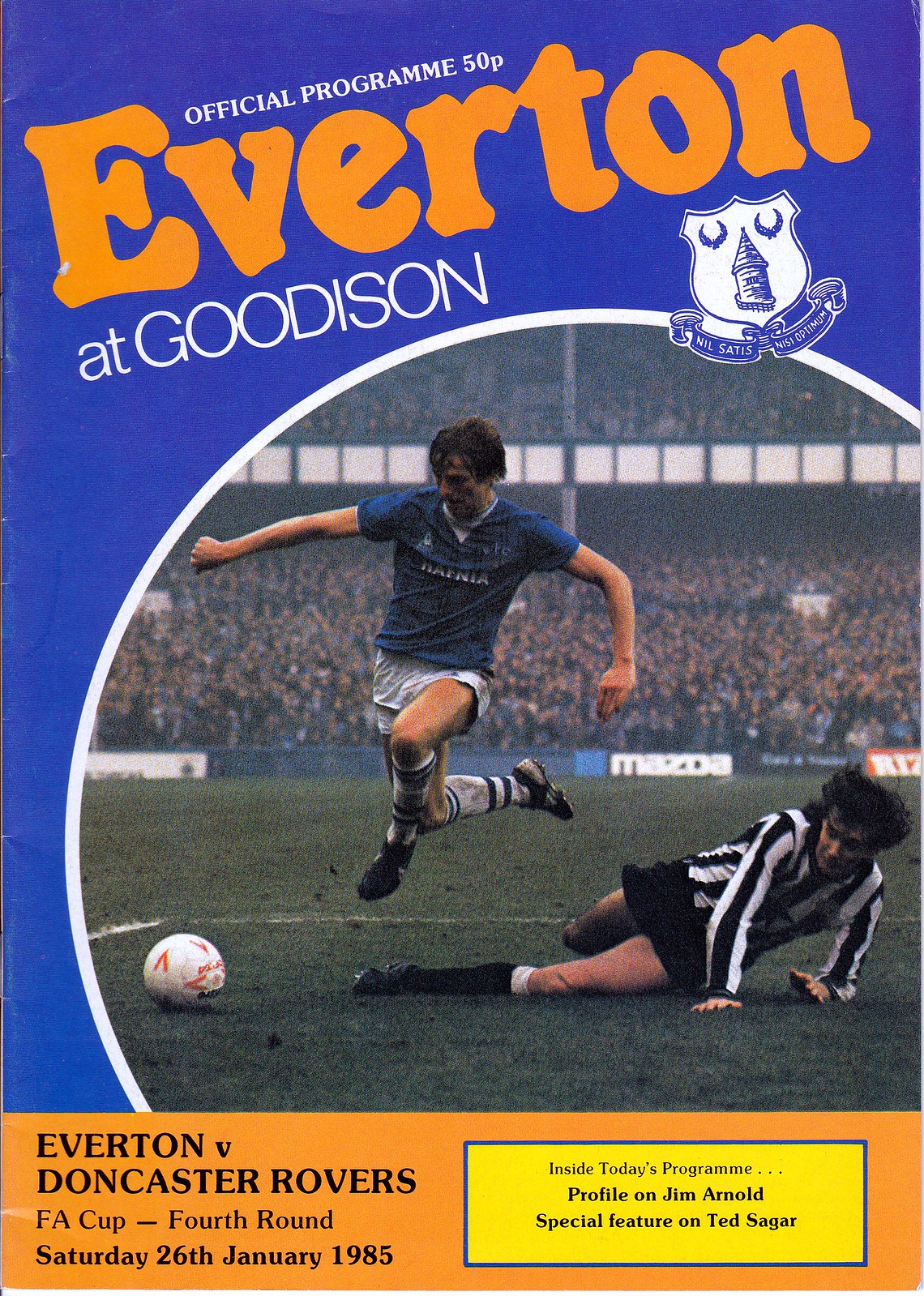The image is the front page of an official program for a soccer game held at Goodison Park, featuring the match between Everton and Doncaster Rovers for the FA Cup fourth round on Saturday, January 26, 1985. The top of the program is dominated by a blue background, with "Everton" written in orange, slanting from bottom left to top right, followed by "at Goodison" in white text. In the middle, there is an action-packed picture of two soccer players: one in a blue jersey and gray shorts, airborne and poised to kick a white soccer ball with red accents; the other, a referee in a black and white striped shirt with black shorts and long black socks, is sprawled on the ground, appearing muddy, as he reaches for the ball. Behind the players is a large, packed stadium. The program also mentions features including a profile on Jim Arnold and a special on Ted Sagar.